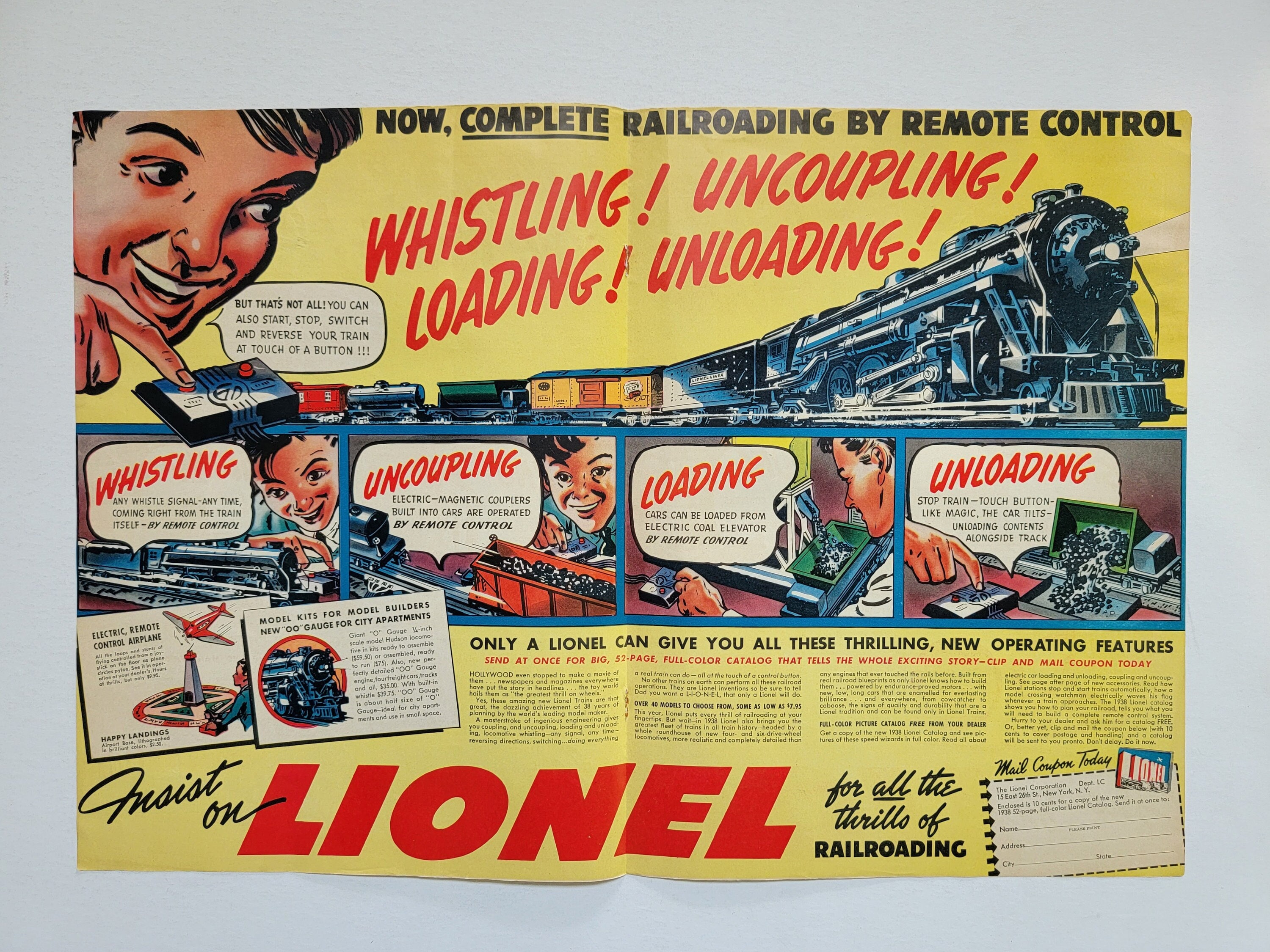The image is a vintage full-page magazine ad for a Lionel remote control train set, depicted in a bright yellow background with a landscape orientation. At the top left, an illustration shows a boy's face, excitedly pressing a remote control button. Bold black text at the top proclaims: "Now Complete Railroading by Remote Control." Below this, in vibrant red, handwritten-style letters, it lists the features: "Whistling, Uncoupling, Loading, Unloading." 

A speech bubble from the boy exclaims additional capabilities: "But that's not all! You can also start, stop, switch, and reverse your train at the touch of a button." Directly beneath, a series of comic book-style panels illustrate these features in detail. The first panel shows a train whistling on command, the second highlights electric magnetic couplers for uncoupling, the third depicts remote-controlled loading from an electric coal elevator, and the fourth demonstrates unloading, where the car tilts to release its contents beside the track.

At the bottom, large text urges: "Insist on Lionel for all the thrills of railroading." Adjacent to this is a mail-in coupon, enhancing the authenticity of the ad's vintage appeal. The ad features a rich palette, including red, light yellow, blue, black, beige, and white, with various sections showcasing different illustrations and text to captivate potential buyers.